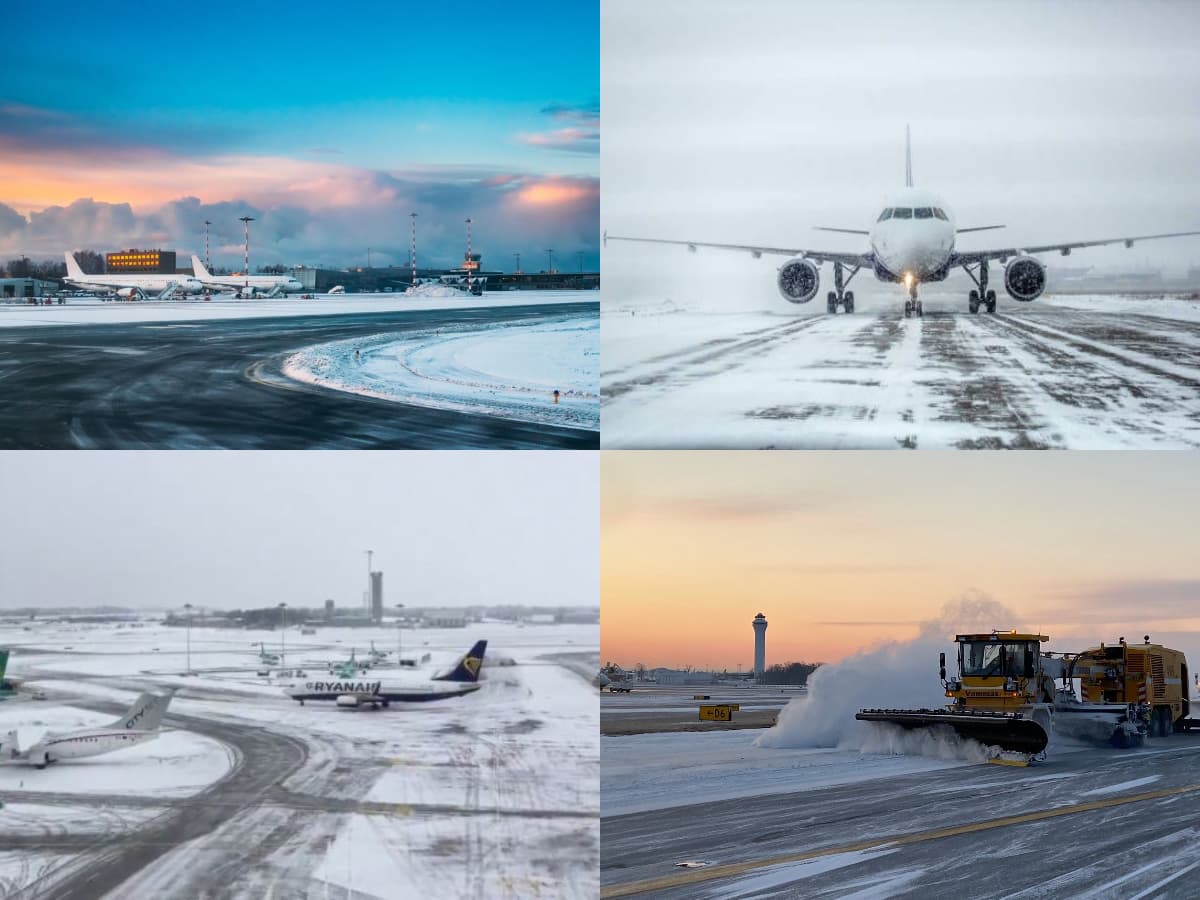This image is a collage of four photographs capturing an airport enveloped in winter conditions. Each photograph highlights different aspects of the snowy environment. 

In the upper left-hand corner, you see a partially cleared runway with two planes resting in the distance under a blue, cloudy sky, suggesting a recent storm. The upper right photograph is a monochrome image featuring a white jet moving towards the viewer on a snow-covered runway, with gray clouds indicating ongoing snowfall. 

The lower left image provides a side view of a snow-blanketed tarmac with a white plane adorned with a blue tail and the Ryanair logo. Off to the side, a smaller plane is parked and a control tower stands in the distance against a gray sky, appearing static in the serene yet cold scene. 

Finally, the lower right-hand photograph focuses on a yellow snowplow actively clearing the runway. The sky above has tinges of golden hues, suggesting either dawn or dusk, as a control tower looms faintly in the background, indicating the gradual return of operational readiness at the airport. 

Together, these images depict the airport grappling with and overcoming the snowy weather.